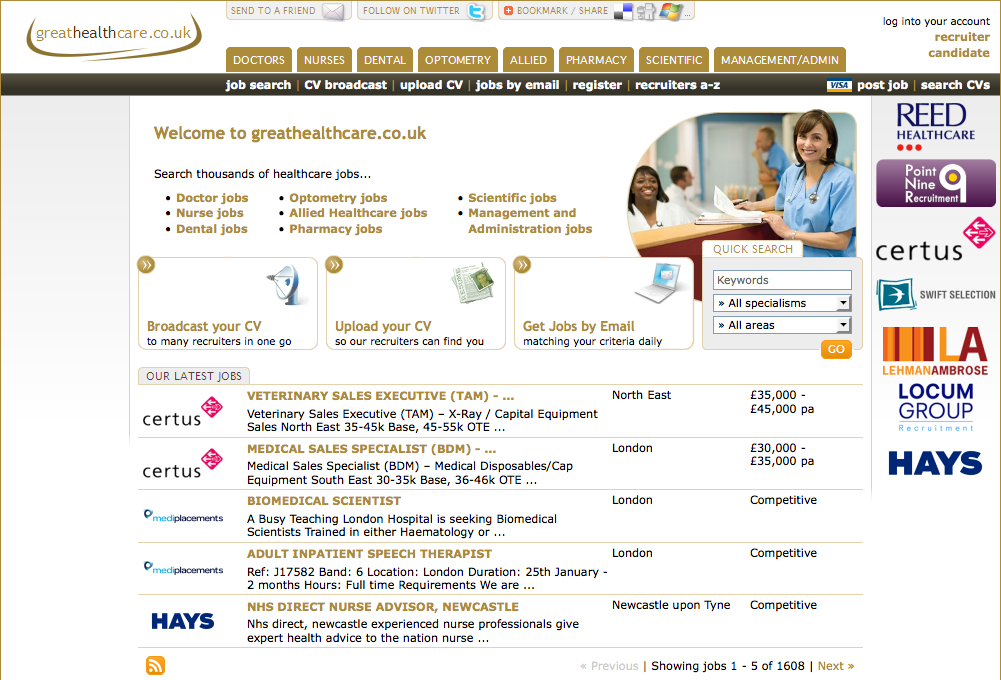This image is a detailed screenshot of a predominantly white website, greathealthcare.co.uk. On the left-hand side, there is a light grey column that fades from pale grey at the top to white at the bottom. At the top of the image, the website's header panel features the site's name, "greathealthcare.co.uk," in a combination of brown and black, encapsulated by two lines forming the base of an oval. 

To the right of the website name are navigation buttons with a gold-brown background and white text. These buttons are labeled: Doctors, Nurses, Dental, Optometry, Allied, Pharmacy, Scientific, and Management/Admin. On the far right side of the navigation bar, there is a "Login to your account" button, with "Recruiter or Candidate" written below it in brown.

A thick black bar runs horizontally across the site, displaying additional options in white text: Job Search, CV Broadcast, Upload CV, Jobs by Email, Register, and Recruiters A-Z. On the far right of this bar, there is a Visa symbol accompanied by the options "Post Job" and "Search CVs."

Below this bar, a white text box contains the greeting "Welcome to greathealthcare.co.uk" in the same browny-gold color. To the right of this text block, there is an image resembling a backwards 'D,' depicting a reception desk with a smiling black woman in a white coat, and another person in scrubs, possibly a nurse or doctor, picking up a piece of paper.

Beneath the welcome message, the site guides users with "Search thousands of healthcare jobs" in black text. The website offers three columns of job categories:
- First column: Doctor Jobs, Nurse Jobs, Dental Jobs
- Second column: Optometry, Allied Healthcare, Pharmacy 
- Third column: Scientific Jobs, Management and Administration

Below these categories, three rectangular blocks outlined in gold provide additional services:
- "Broadcast your CV" with a satellite dish icon
- "Upload your CV" with a stack of papers icon
- "Get jobs by email" with a laptop icon

Adjacent to these blocks is a Quick Search feature where users can input keywords, specialisms, and areas. 

Further down, under "Our Latest Jobs," the website displays job listings in four columns:
- Logos and names of the hiring companies (e.g., Certus, Med Placements, Hayes)
- Job titles and brief descriptions
- Job locations
- Annual salaries

At the bottom of these listings, the page indicates that it is showing jobs 1 to 5 out of 1,608, along with a "Next" button for navigation. 

The right-hand column of the website features adverts for healthcare suppliers such as Reed Healthcare, Point Nine Recruitment, Certus, Swift Selection, Lehman Ambrose, Locum Group, and Hayes.